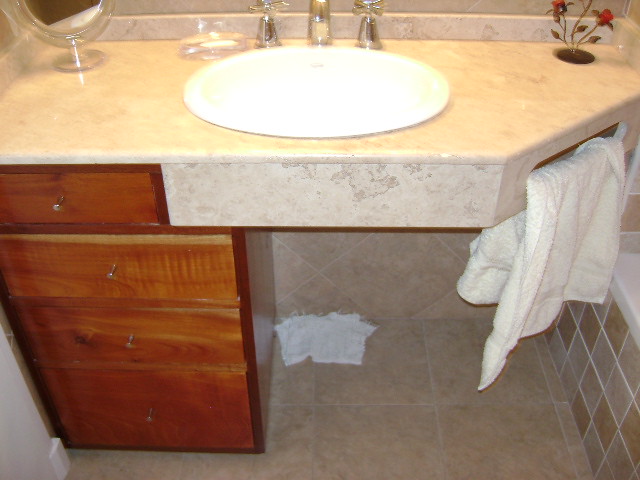Here's a detailed caption based on the provided description, with an emphasis on clarity and thoroughness:

---

The image showcases a bathroom sink area, characterized by an elegant and earthy color scheme. The wall behind the sink features tan-colored tiles, accented with a beige trim along the top portion of the counter. The countertop displays a blend of light tan, brown, and grayish colors, presenting a natural stone-like finish. 

To the left of the sink, a brown cabinet is visible, equipped with shiny, silver round knobs for the drawers. On the right side of the counter, a towel holder is mounted, providing easy access to a white towel that is positioned beneath the countertop, partially draped on the floor. The wall beneath the counter is adorned with more of the beige tile, while the same tiling extends onto the floor itself.

Adjacent to the bathtub, to the right, there is a display of brown and tan-colored tiles. A clear or silver-framed mirror is situated on the left side above the counter, reflecting the soft ambient light of the room. 

The centrally positioned white sink is complemented by chrome faucets and handles, giving it a modern touch. Adding a splash of color and life to the space, a small potted plant with red and green flowers is placed on the right side of the countertop, next to the sink, enhancing the overall aesthetic of the bathroom.

---